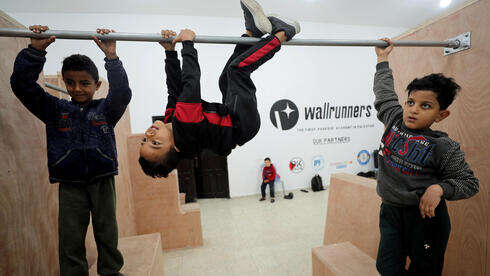This photograph captures an indoor play area, seemingly a warehouse converted into a children's playground. The background showcases a white wall adorned with signage, prominently featuring a circle with a white star, a line, and the words "Wall Runners", accompanied by additional, unreadable text. A person sits on a chair near this wall. 

In the foreground, the main scene unfolds around a metal bar, horizontally affixed between large wooden structures, possibly serving as support. The floor beneath is smooth and yellow. There are three boys interacting with the bar, all dressed in winter clothes, including jackets and pants.

- On the left, the first boy, dressed in a blue jacket and light green pants, stands on a wooden block. His hands grip the bar as he faces slightly to the left.
- The boy in the middle hangs upside down, using both his hands and feet to cling to the bar. He is garbed in a black outfit with red stripes.
- The boy on the right, wearing a sweater with blue, red, and white writing and dark pants, reaches up to grasp the bar with one hand. Behind him, a light-colored bench is partially visible, suggesting he might also be standing on an elevated surface.

This lively scene of playful children is set against an engaging backdrop, indicating a well-designed space for active play.